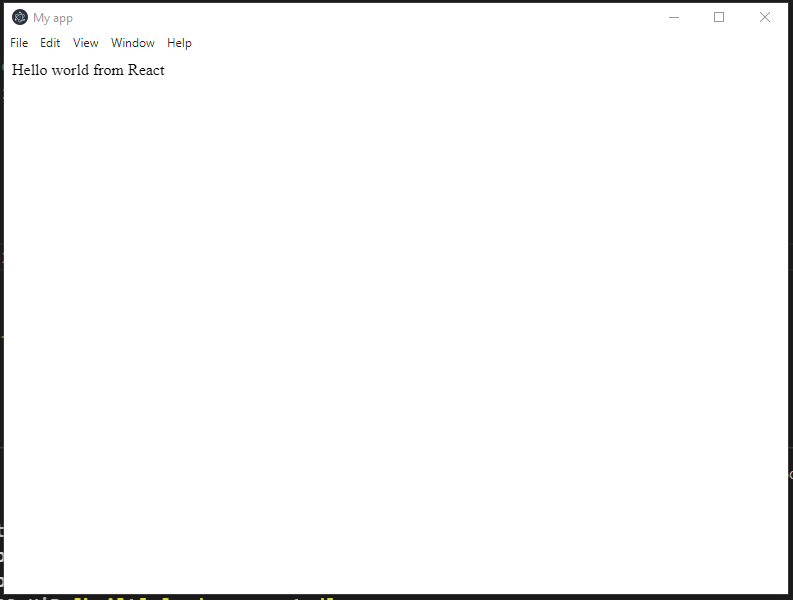The image displays a square interface with a black border surrounding a white interior. In the top left corner, there's a circular icon labeled "My App." To the right of the icon are three buttons: minimize, maximize, and close (X). Directly below the "My App" label is a horizontal menu bar with the following options listed in black text: "File," "Edit," "View," "Window," and "Help." Beneath this menu bar, the text "Hello World from React" is prominently displayed. The majority of the square's background is plain white, giving it a minimalistic appearance. Every word in the image is clearly spelled out, further emphasizing the simplicity and clarity of the interface design.